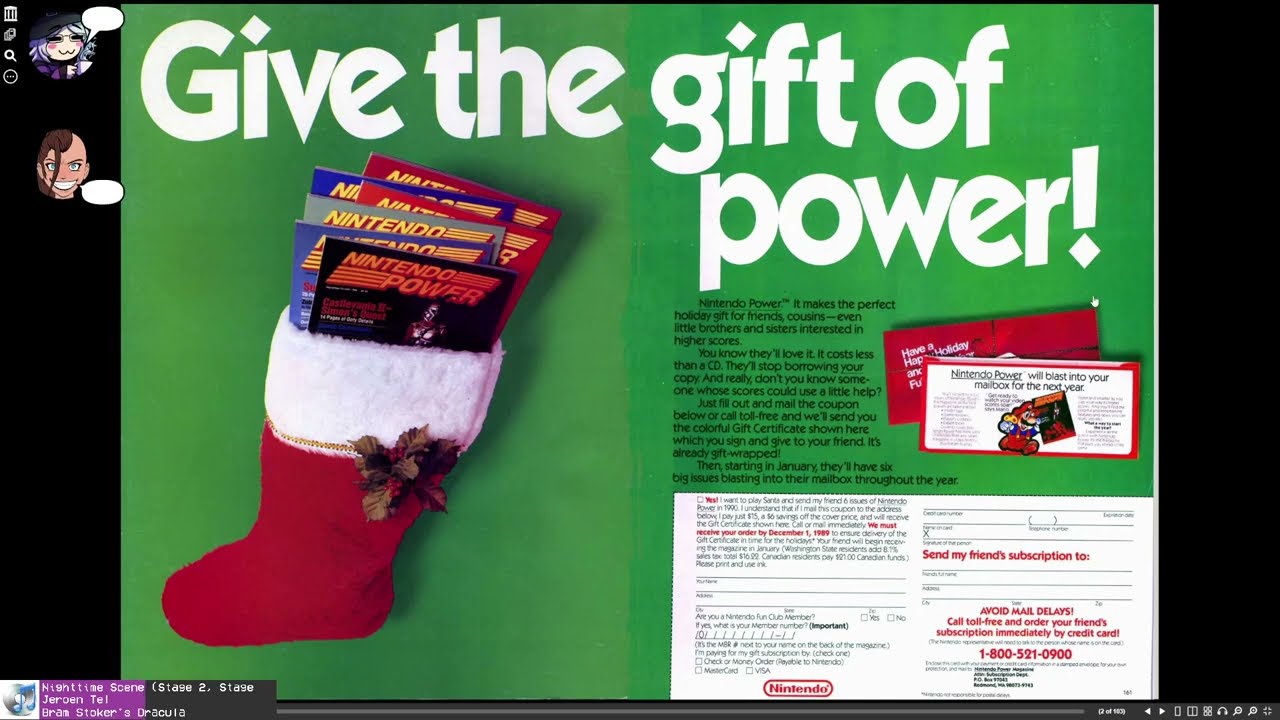This advertisement, reminiscent of an old Nintendo Power Magazine ad, showcases a bright green background with bold white text at the top that reads, "Give the Gift of Power." The ad features a festive red and white Christmas stocking with a fluffy white top, adorned with a gold trim, overflowing with Nintendo Power magazines. The promotion is centered on gifting the subscription, highlighting it as the perfect holiday gift for friends, cousins, and younger siblings who are eager to improve their gaming scores. The ad suggests that giving Nintendo Power is a cost-effective present that recipients will appreciate, urging readers to stop sharing their own copies. Additional details include a black banner with various icons in the upper left corner and two avatars with speech bubbles, suggesting a conversational or live chat format. In the lower right corner of the image, there is a white rectangular area providing space to fill out personal information such as name, phone number, and possibly credit card details to order the magazine. A toll-free 1-800 phone number is also provided for easy subscription.